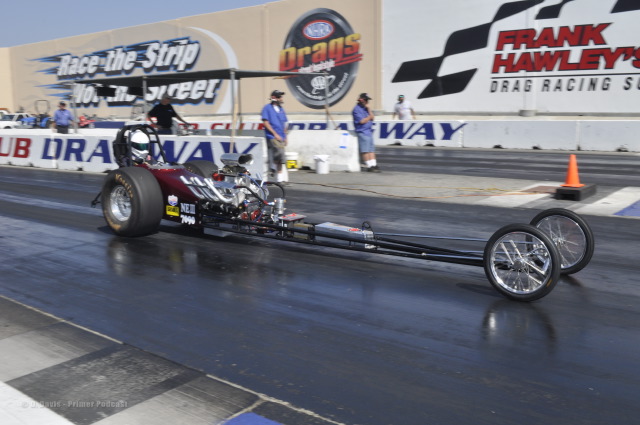The image captures an exhilarating moment at a drag race show featuring a striking drag race car poised on a black, shiny, reflective tarmac. The drag race car, which is not intended for conventional driving, is notably long with an exposed silver engine situated between two elongated metal poles connected to two very small wagon wheel-type tires in the front. Behind the engine is a compact driver's seat encapsulated by a robust black roll cage, flanked by massive racing tires with prominent yellow lettering on their sides. In the distance, various team members bustle around the pit stop area. The backdrop is dominated by a large wall adorned with multiple logos and signs, including one on the right that reads "Frank Hawley's Drag Racing Show." Additional details such as safety cones are also visible, adding to the authenticity and typical atmosphere of a high-octane drag race event.